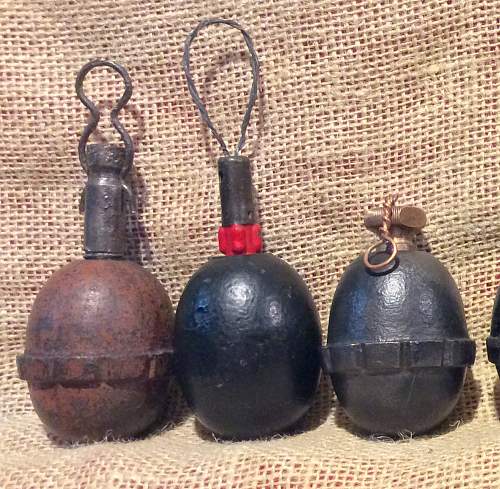The image depicts a close-up view of three heavy, cast iron objects resembling old-style grenades or lantern bases, placed against a coarse, burlap-like fabric background. Each object is primarily oval-shaped with distinct cylindrical protrusions and unique top fittings. The leftmost object is a rusty brown color with extruded metal segments ending in a rounded hook at the top. The middle one is glossy black, smooth, and features a red base near the neck, with a rounded hook above it. The rightmost object is a dark gray with four metal segments jutting out just below the midpoint, topped by a mushroom-shaped cap with a brass wire loop dangling over the edge. The metal surfaces and varied fittings suggest they might have held lampshades or could potentially be antique military items repurposed as decorative pieces.